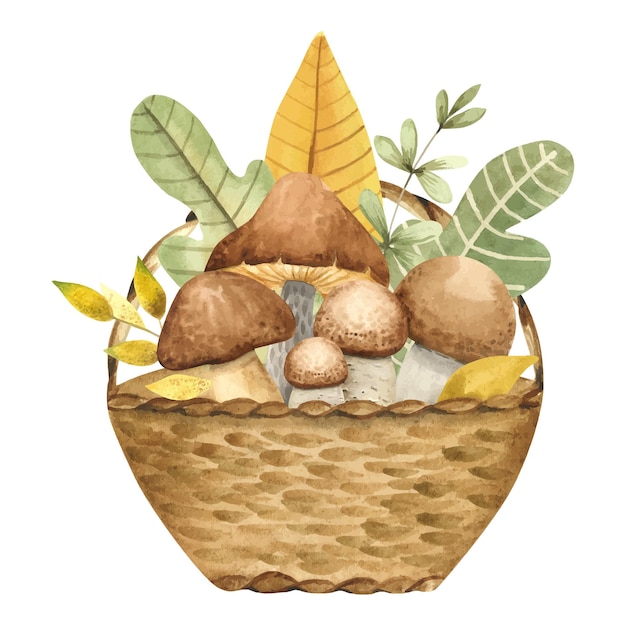The image is a detailed painting of a woven wicker basket with various brown and tan shades, featuring a large, rounded handle arching over the top. Inside the basket are five distinct mushrooms. The first two mushrooms have darker brown, rounded caps with white undersides and grayish-white stalks. The other three mushrooms have lighter brown tops, with thicker, whiter stalks. Surrounding the mushrooms are a mix of large and small leaves, some of which are green while others are golden yellow. The leaves exhibit rich green veining, adding texture. The entire composition predominantly features earthy tones, including greens, browns, and golds, creating a harmonious and naturalistic scene.